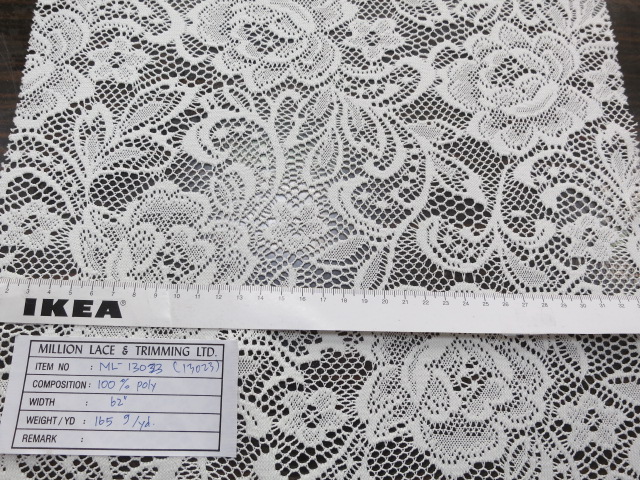This image is a detailed close-up color photograph of a piece of white lace fabric laid against a black background. The perspective looks directly down onto the fabric, showcasing its intricate knitted flower patterns, complete with leaves and connecting stems. The fabric is being measured with a white IKEA measuring tape that spans horizontally across the bottom third of the image, with its black markings and bold "IKEA" logo clearly visible on the bottom left. Below the measuring tape, there is a white tag labeled "MILLION LACE & TRIMMING LIMITED," followed by handwritten details in blue ink mentioning item number ML130313, a composition of 100% poly, a width of 62 inches, and a weight of 165 nine/yards. The tag also includes a blank section for remarks. The photograph, with its landscape orientation and the sharp focus on the lace and measuring tape, suggests a realistic, product photography style.